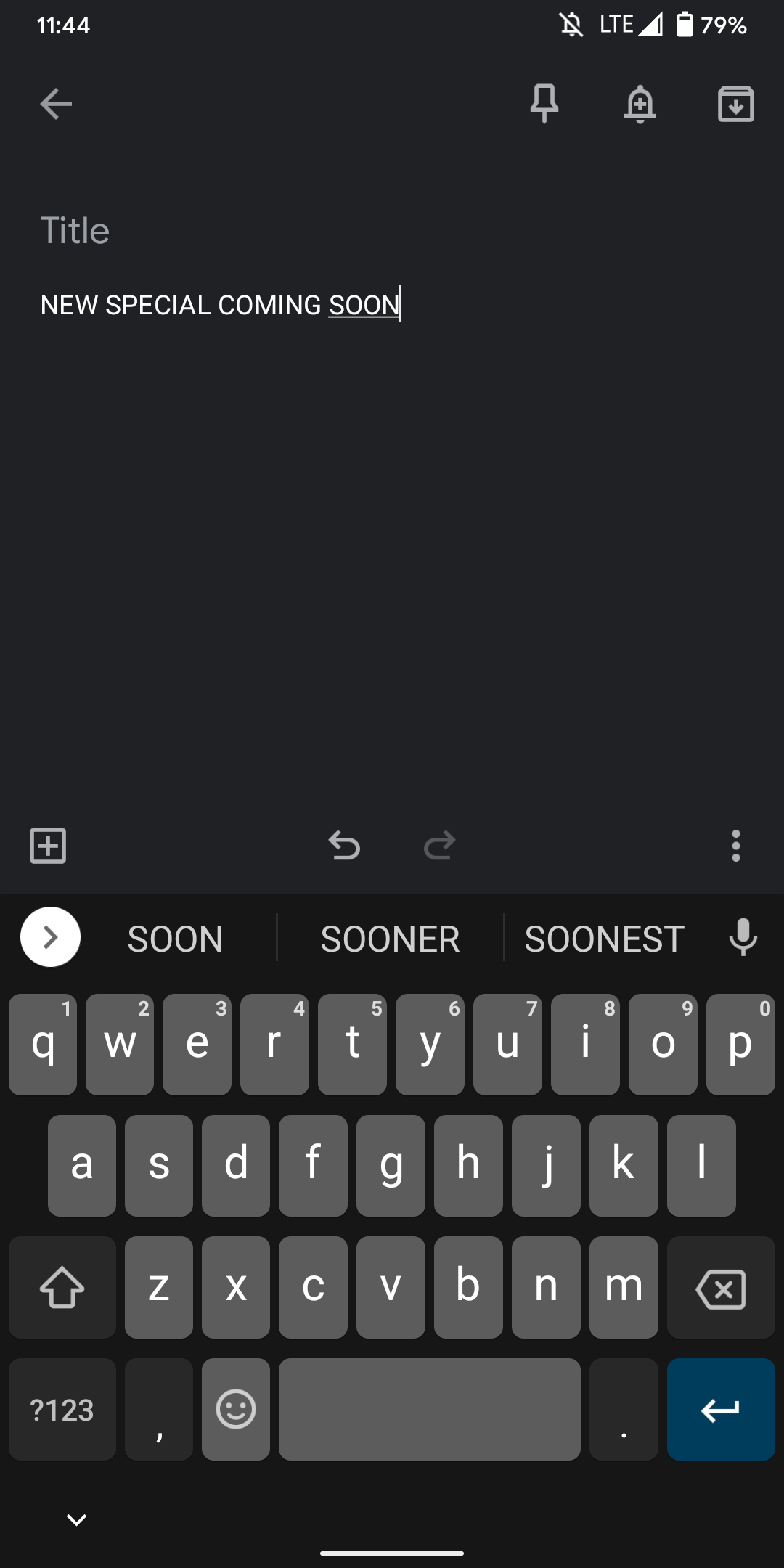A detailed descriptive caption for the image could be:

"A screenshot of a cell phone's notepad in night mode, featuring a black background with dimmed elements for nighttime usability. At the top left corner, there is a gray back arrow icon. To its right are icons for pinning notes, setting reminders, and downloading content. The header displays the word 'Title' in dark gray font. Below this header, a small white text in all caps reads 'NEW SPECIAL COMING SOON.' The phone's keyboard is visible at the bottom, with a bright blue "Enter" button on the bottom right. Above the keyboard, text suggestions for the word 'soon' are displayed, including 'soon,' 'sooner,' and 'soonest.' Additionally, there is a box containing a plus sign on the top left, and undo/redo arrows in the center. In the top right corner of the screenshot, status icons indicate that the phone's alarm is off, it is connected to LTE with a strong signal, the battery is at 79%, and the battery icon is visible."